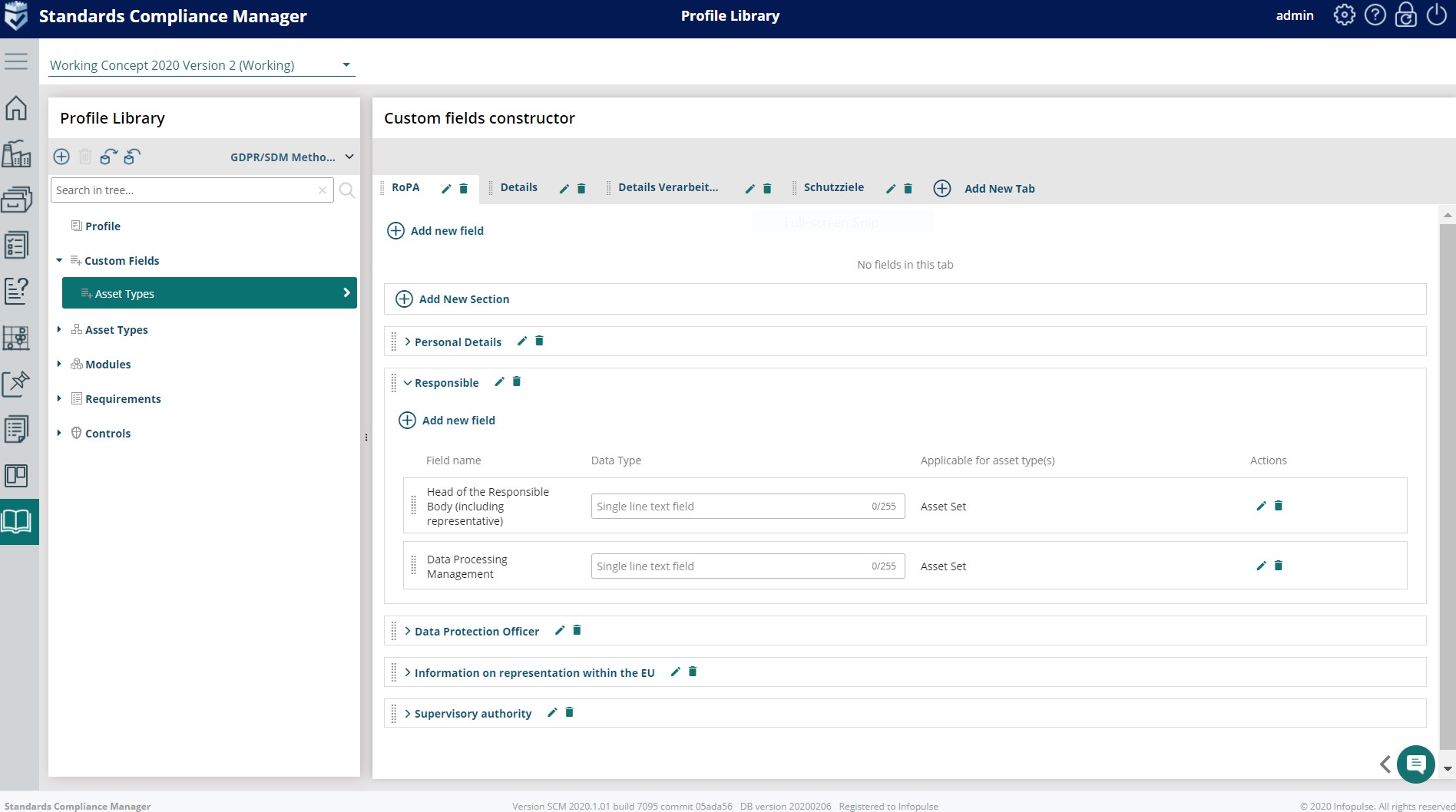The screenshot depicts a comprehensive interface of the "Standards Compliance Manager" dashboard. Positioned against a dark blue background, the title "Standards Compliance Manager" is displayed in white font at the upper corner. At the very top, a prominent dark blue border encompasses the page, while centrally located within this border, the phrase "Profile Library" is highlighted.

On the left side of the screen, the navigation panel lists several options, beginning with "Admin" and including an icon resembling a question mark, likely indicating a help or support section. The primary background of the page is white, accentuating a sidebar on the left.

At the top of this sidebar, written in a very light green shade, is "Working Concept 2020 Version 2" with "Working" noted in parentheses. Below this, "Profile Library" is denoted in black font. The sidebar further enumerates a vertical list of menu items in black text: "Profile," "Custom Fields," "Account Types" (highlighted with a green box), "Asset Types," "Modules," "Requirements," and "Controls."

Dominating approximately three-quarters of the middle section of the screen, the main content area features a header in white font reading "Custom Fields Constructor." Below this header, there are four tab options; the first tab, labeled "R0PA," is active, while the remaining three tabs appear gray and include titles such as "Details" and additional text in German that is partially obscured.

Beneath these tabs, the section is set for configuration tasks, situated on a white background. Several options are present within this zone, including an "Add New Section" button accompanied by a circular icon with a plus sign on its left side, suggesting that clicking it would likely reveal additional configuration choices.